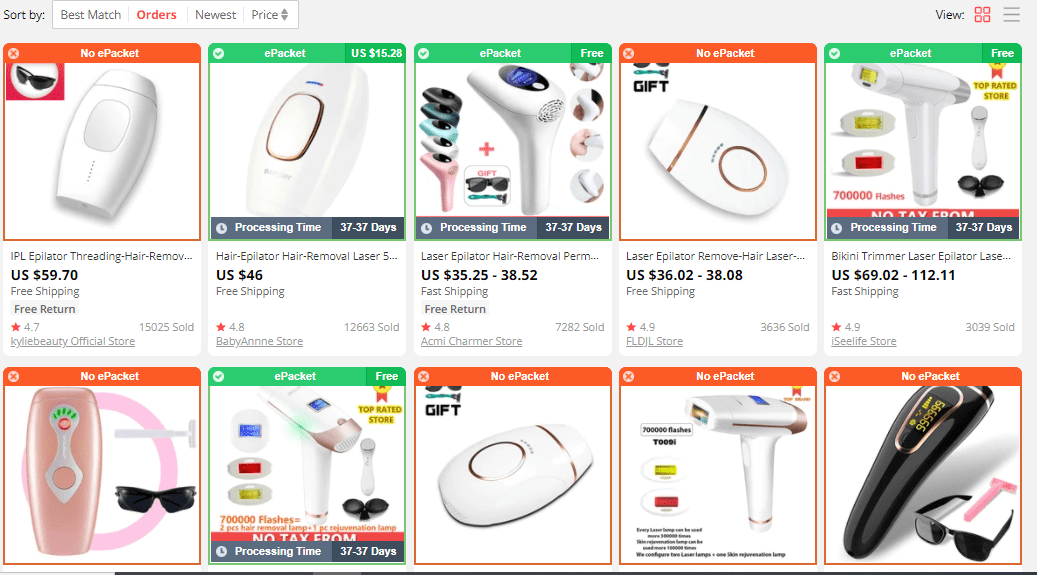The image showcases an online shopping page with a clean white background. The layout includes ten distinct purchase options, each illustrated in color. At the top of the page, there are five selectable sections for modifying the displayed products: "Sort By," "Best Match," "Orders," "Newest," and "Price." Adjacent to these tabs are up and down arrows for further sorting options. In the far left corner, there are additional page customization tools. A "View" option is presented next to an icon featuring four mini squares within a larger square, likely indicating different layout choices. Next to this, another icon with three horizontal stacked lines possibly offers more detailed settings or menu options. Each of the ten product windows is highlighted in either orange or green: orange indicating items without e-packet shipping and green for those with e-packet shipping. The displayed products are various types of hair removal tools, including hair trimmers, epilators, and other similar devices from different manufacturers and models.